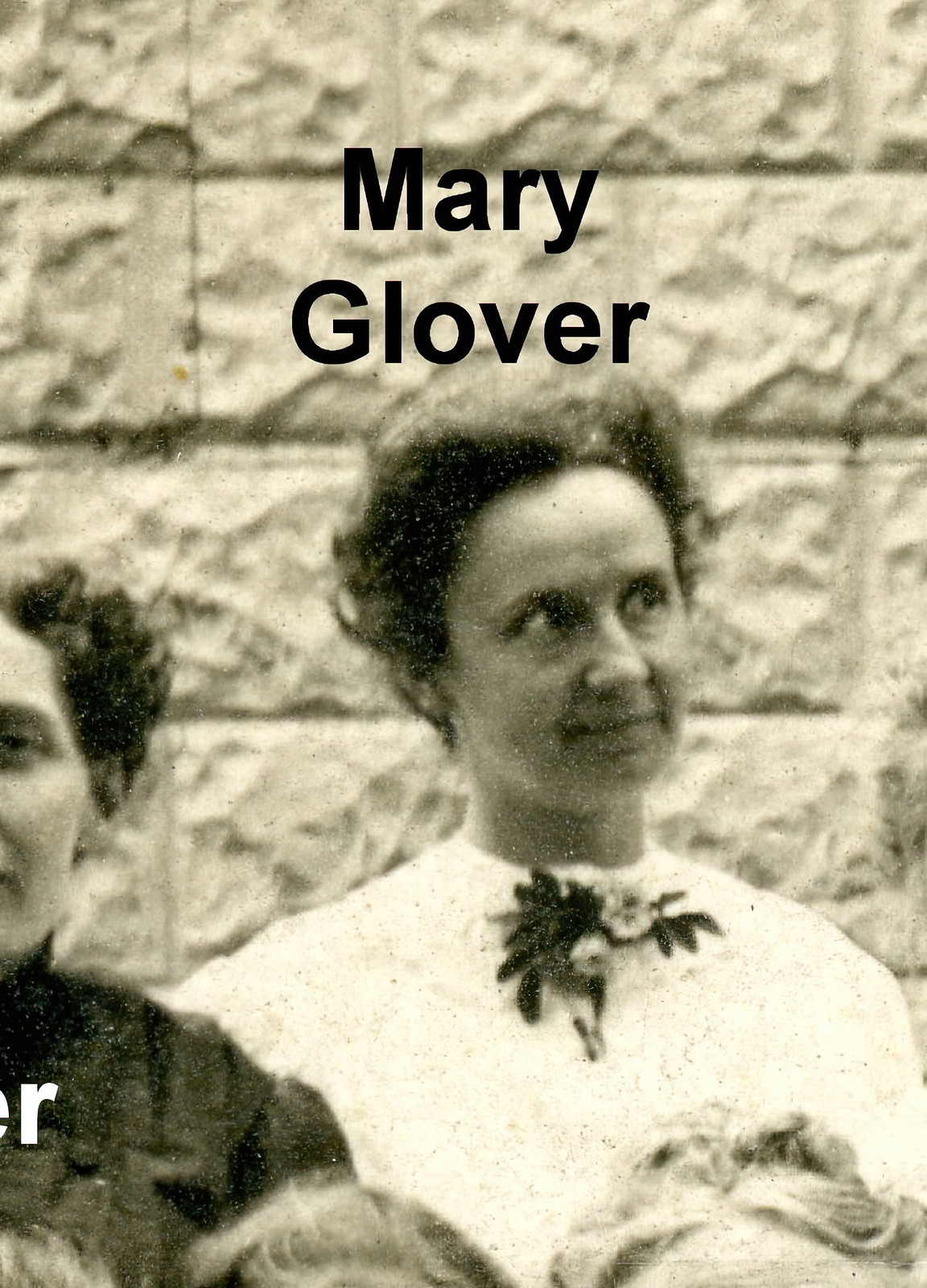This vintage black and white photograph, likely from the early 1900s, features a Caucasian woman with short, dark, frizzy hair styled in a bun. She is elegantly dressed in a high-necked, long-sleeved white blouse adorned with a floral accessory at the collar. The woman is facing the camera but gazes upwards toward her right. She stands before a high, light-colored brick or stone wall, above which the name "Mary Glover" is inscribed in bold black letters. The image's foreground is populated by the tops of the heads of three other women, with another partially visible woman standing to her left, who also has dark, frizzy hair and wears a high-necked blouse of a darker shade. The photograph is grainy and shows signs of age, adding to its historical charm and classical appearance.